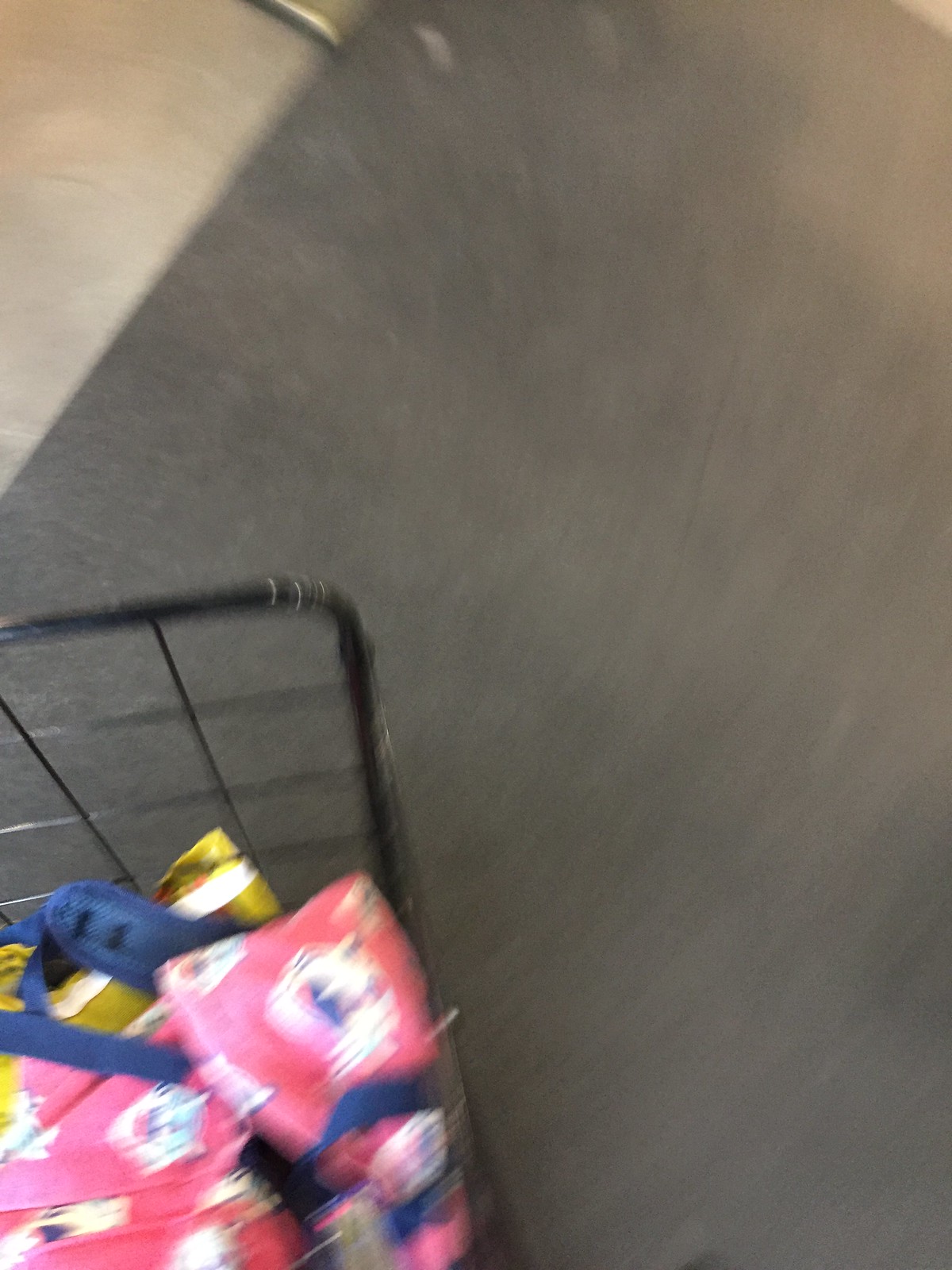This color image, likely taken overhead with a cell phone, is a bit blurry and exhibits a swirling effect, suggesting the camera was in motion. The main subject is a black metal shopping cart positioned in the bottom left corner of the frame. The cart's design features a grid-like pattern formed by intersecting vertical and horizontal lines. Inside the cart, there is a bright pink bag or backpack with blue straps, accompanied by a yellow package with a white banner on top. Additionally, there are various containers in shades of pink, white, and blue dispersed throughout the cart. The background of the image is a mix of gray asphalt and a lighter, off-white or tan area at the top left, with a touch of gold.